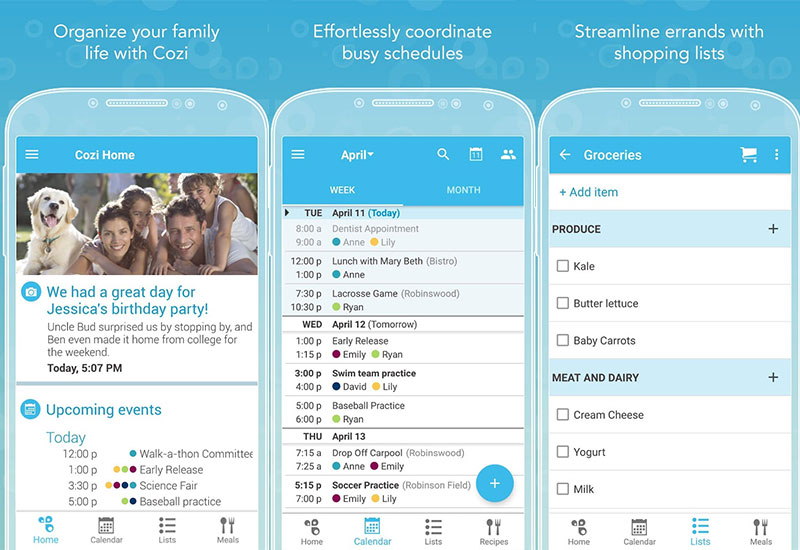The image is a detailed screenshot of an app interface divided into three distinct sections, each highlighting a unique feature of the app designed to enhance family organization.

1. **Organize Your Family Life with Cozy**: This section features a blue header bar and includes an image of a cheerful family consisting of a man, a woman, two kids, and a dog positioned on the left side. Below this image, a headline reads, "We had a great day for Jessica's birthday party," setting a warm, personal tone. The section also highlights upcoming events with text displayed in blue, suggesting a focus on family activities and planning.

2. **Effortlessly Coordinate Busy Schedules**: The second section emphasizes the app's calendar functionality. It displays a weekly calendar view, likely showing different family members' schedules. This section reiterates the app's goal of helping users manage and coordinate various activities seamlessly.

3. **Streamline Errands with Shopping Lists**: In this section, the app showcases its capability to organize shopping needs. A grocery list appears on the screen with items such as kale, butter, lettuce, and baby carrots, each accompanied by a checkmark indicating completed purchases. This feature aims to simplify grocery shopping and ensure nothing is forgotten.

Each section is supported by a visual representation displayed on a smartphone, reinforcing the app's user-friendly design and practical use in daily life.